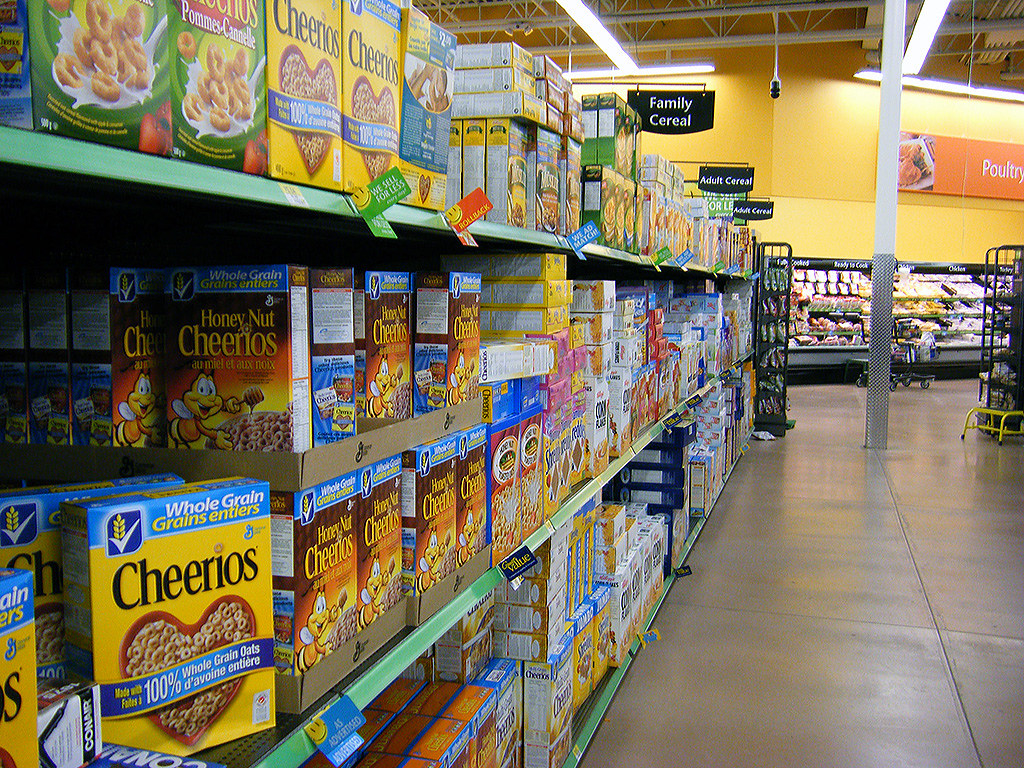This digital photograph taken indoors in what appears to be a Walmart depicts an aisle primarily filled with cereal. The shot is taken from the end of the aisle, looking straight down. On the right side of the photo, a bright yellow wall and a poultry sign in orange are visible, along with metal ceiling trusses painted white. Below, there are black open-air refrigerators with indiscernible white writing. The floor is a nice gray concrete.

The left side of the image is dominated by a three-tiered shelf of cereals. The top shelf prominently features yellow boxes of Cheerios, with darker orange and light orange boxes of Honey Nut Cheerios beside them. The middle shelf also contains Cheerios and assorted Honey Nut Cheerios. The bottom shelf's contents are not visible from this angle. Various other cereal boxes in blue, red, and green can be seen further down the aisle. 

Three black signs with white letters hang above the shelves, labeling the sections: one closest to the viewer reads "Family Cereal," followed by two signs indicating "Adult Cereal." In the background, there are racks of meat in a refrigerated section, partially obstructed by a cart and a pole. 

Overall, the image provides a clear and detailed view of the store's neatly organized cereal aisle, with additional glimpses of the store's signage, structure, and layout.